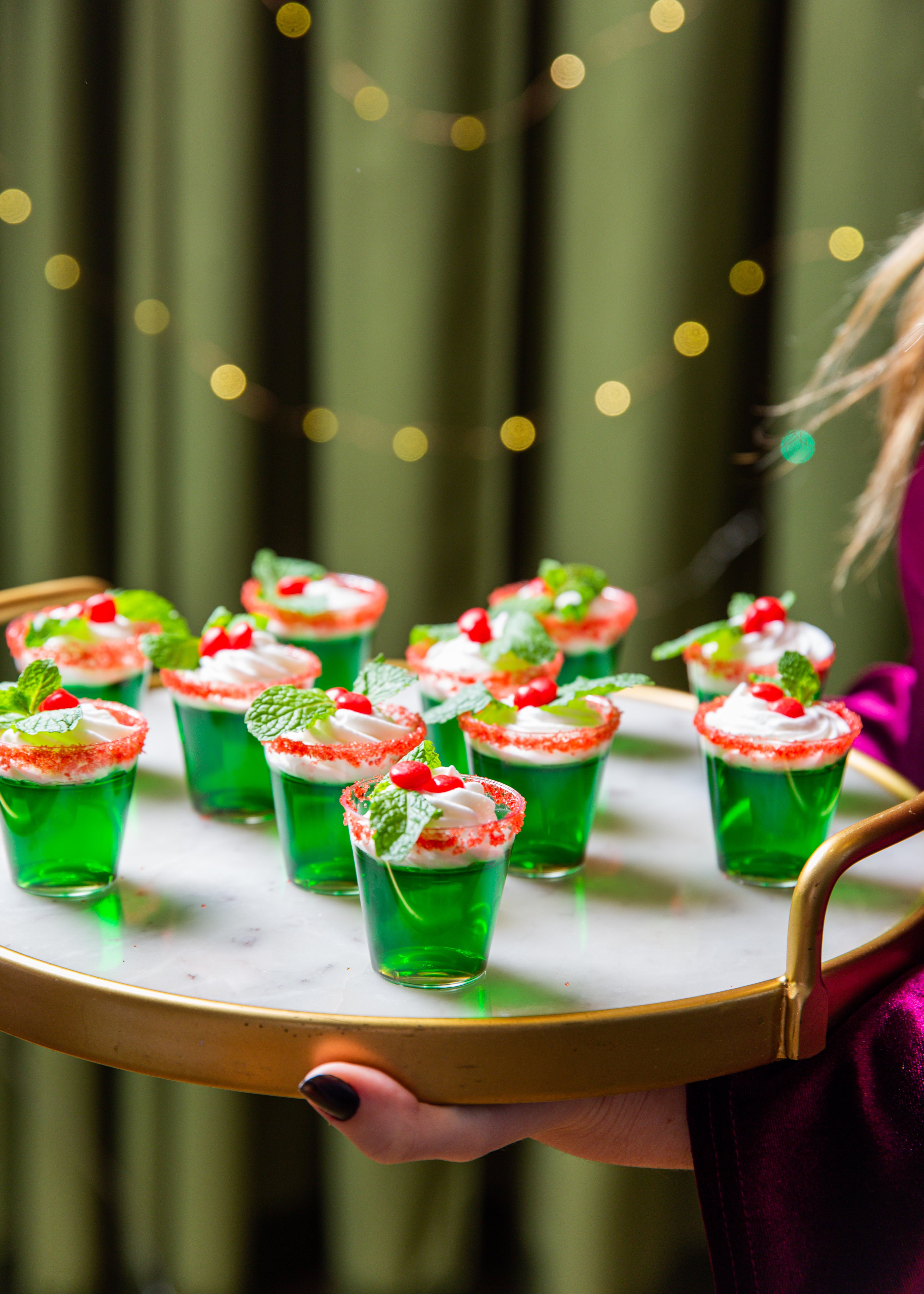In this portrait-layout photograph, a Caucasian woman with blonde hair and black nail polish is carrying a white tray adorned with gold handles and a gold border. The tray holds exactly 11 green jello shots, each topped with white whipped cream, two red cherries, and a green mint leaf, with a red sugar or salt rim around the top of each shot glass. Her thumb, slightly peeking from beneath the tray, reveals her black-painted nails. The background is blurred but features a green draping with sparkling twinkle lights, adding a festive, almost magical ambiance to the scene. The woman is dressed in a purple long-sleeve shirt, contributing to the overall cozy yet elegant atmosphere of the photograph.